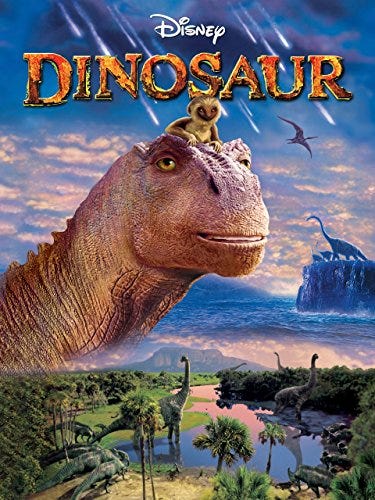The image is a vibrant and detailed poster for the Disney movie "Dinosaur." Dominating the foreground is the head and neck of a large, brownish dinosaur, akin to a Brontosaurus, with a serene expression as it looks toward the viewer. Perched on its head is a small, white-furred creature, resembling a monkey or koala, with strikingly colorful eyes. Surrounding this central character is an expansive, lush green landscape featuring tall palms and a river meandering through the dense forest. Several other Brontosaurus-type dinosaurs can be seen roaming the scenery, adding depth and a sense of community. In the background, a massive body of water stretches out, blending into a mountainous area from which more dinosaurs peak. The day sky unfolds dramatically with meteorites streaming down, narrowly missing a pterodactyl that soars through the air. The entire scene blends elements of still photography and painting, creating a dynamic and engaging composition. At the top of the image, the title "Dinosaur" is prominently displayed, along with the iconic Disney logo, tying the visual storytelling together.